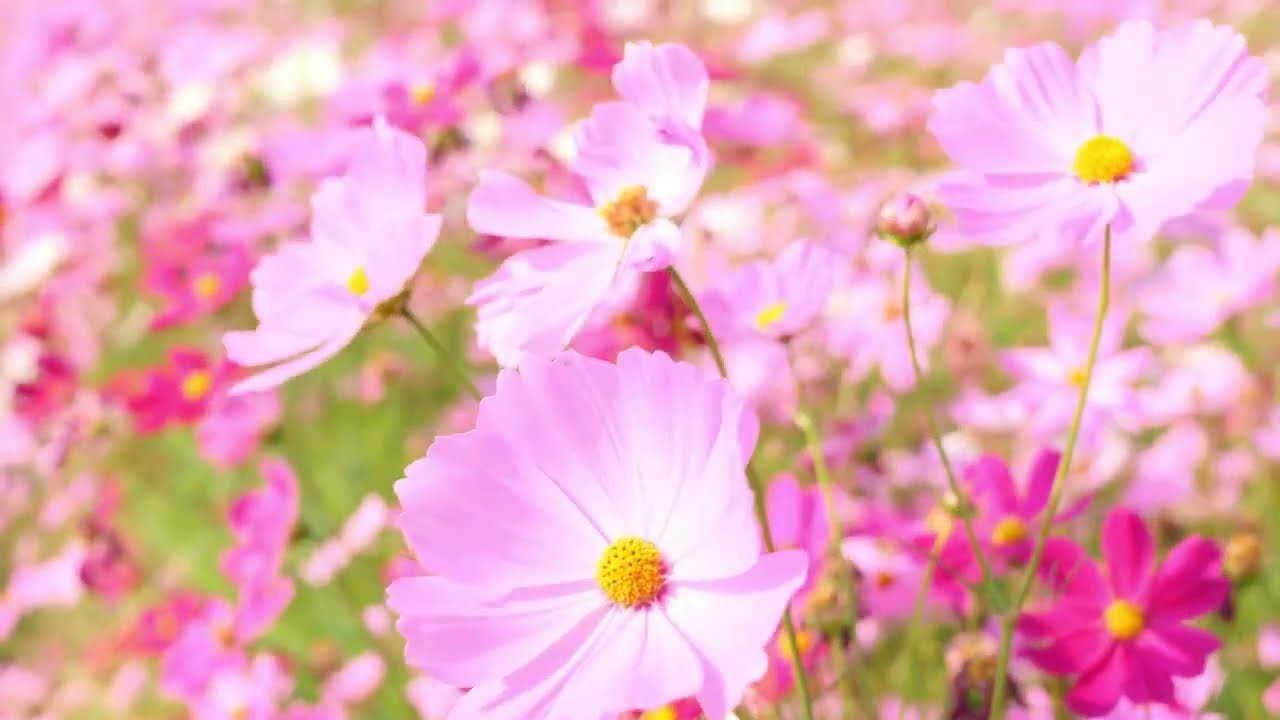The image captures a vibrant outdoor scene in a meadow or field filled with an array of blooming flowers. Dominating the foreground are striking flowers with petals that transition from white at the base to a delicate pinkish-purple at the tips, complemented by a vivid yellow center. These flowers are anchored by long green stems and surrounded by lush green leaves. Interspersed among them are hot pink carnations with similarly bright yellow centers. The background is artistically blurred, offering a glimpse of more flowers in various shades of light pink, darker pink, and white, hinting at a colorful expanse. Some buds are still getting ready to blossom, adding to the sense of a lively, blooming field captured in the natural daylight. The overall composition suggests a serene, natural setting, perhaps a garden or park, meticulously photographed to highlight the beauty and diversity of the floral display.